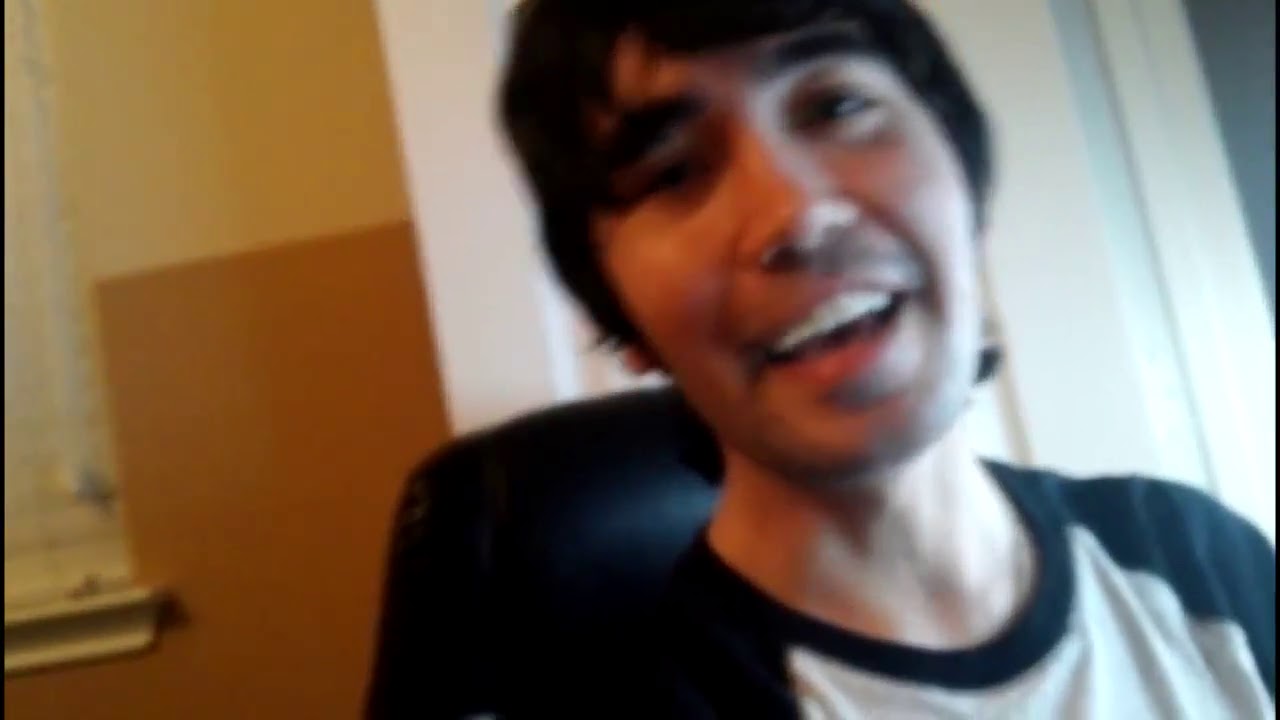The image is a slightly out-of-focus photograph, tilted a few degrees to the left, capturing a close-up of a young man, around 18 or 19 years old, sitting in a black chair. He has dark, short but not very short hair, and bushy eyebrows. His head is tilted a bit to the left, and he is smiling with his mouth open as if he is about to speak or in the middle of talking. He is wearing a white t-shirt with black sleeves and a black collar. The background shows a room with an open white door and a two-toned wall—brown wooden paneling or golden at the bottom and tan or yellowish at the top. On the left side of the image, there is a window with white blinds drawn shut, and in the lower left-hand corner, there is an out-of-focus object that appears to be a white faucet, possibly indicating a sink nearby.